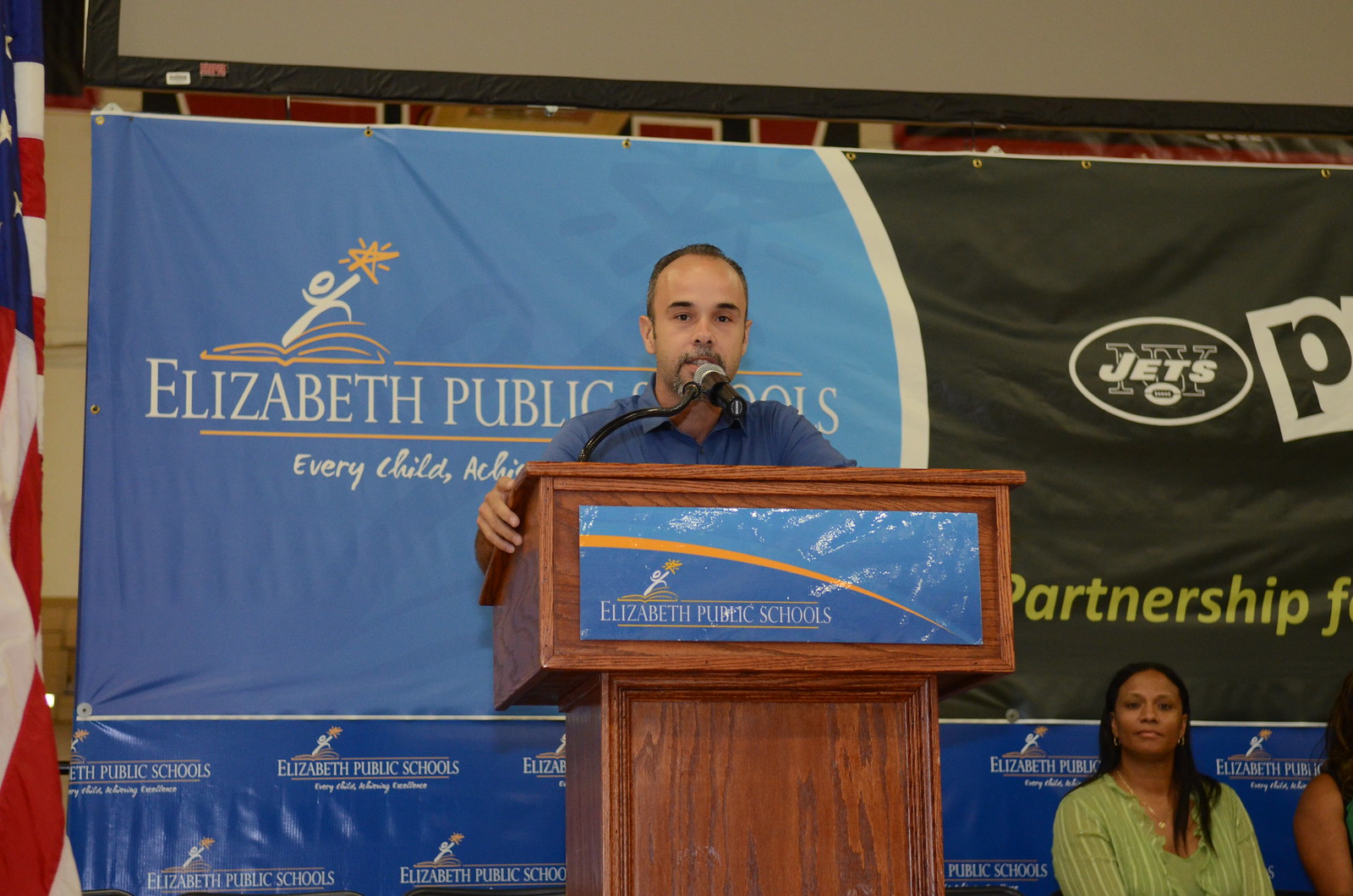This vibrant full-color photograph captures an indoor event likely taking place in a school or assembly hall. On the far left, there is a partial view of an American flag. At the center stands a man at a wooden lectern adorned with a blue sign that reads "Elizabeth Public Schools," speaking into a microphone. Behind him stretches a large banner, partially obscured by the speaker, displaying "Elizabeth Public Schools" and "Every Child." A green segment of the banner features the New York Jets logo, indicating a partnership between the Jets and the public school. To the left of the gentleman, the words "partnership" can be seen above the head of a seated woman. This woman is an African American with long black hair, dressed in a lime green shirt that has a low v-neck. She is looking directly at the camera. Another individual, partially visible, is seated adjacent to her. The man at the lectern appears to be of Mexican-Cuban descent and is engaged in delivering a speech, contributing to the formal and collaborative atmosphere of the event.